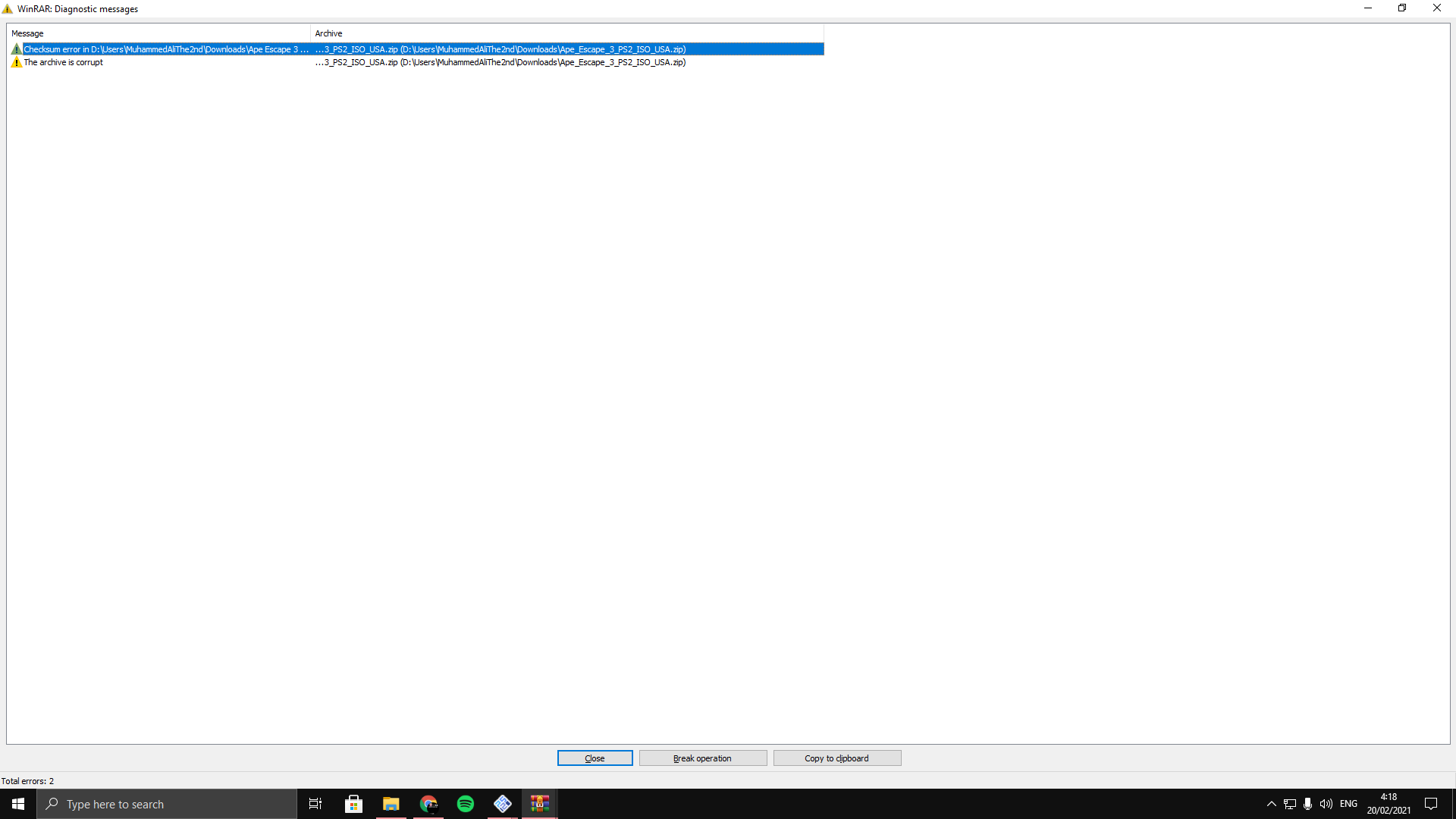A screenshot displays a diagnostic message from WinRar. In the upper right corner, a yellow yield icon with an exclamation point warns of a checksum error related to an ISO file being opened, highlighting the inadvisability of compressing an already semi-compressed format. Below, an error message indicates that the archive is corrupt. The bottom of the screenshot features a black Windows 10 taskbar. On the left, icons for Windows Insignia, Windows Search, Windows Store, File Explorer, Chrome, Spotify, an unspecified app, and WinRar are visible. The right side includes icons for monitor connection, sound settings, English options, and a microphone. Notifications are turned off, and the system time is set to a European format, displaying "18:04, 2021." A notification pop-up in the bottom right corner shows no active notifications.